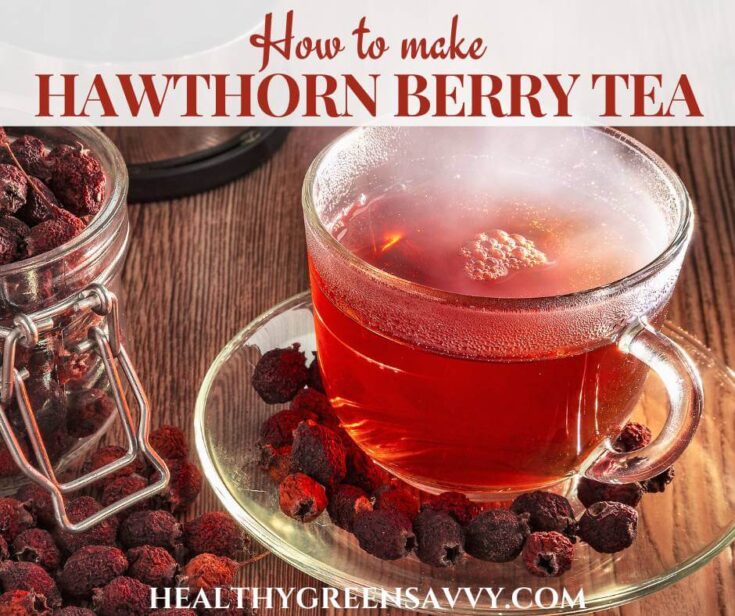The image is a detailed color photograph in landscape orientation, seemingly taken from a food blog or an advertisement for making hawthorn berry tea. At the top of the image, there is a semi-transparent white banner with a maroon-colored headline that reads, "How to Make Hawthorn Berry Tea." Below the headline, centrally positioned, is a clear glass cup on a matching glass saucer. The cup, showing an inviting handle facing the right, contains an amber-colored tea that appears hot and steamy, with a slight foam on the surface. Nestled on the saucer and scattered on the wooden table surface are several red hawthorn berries. To the left of the cup is an open clear glass jar with a silver closure, filled with additional hawthorn berries. The wooden table has a dark, vertically grained texture, providing a rustic background for the tea setup. At the bottom of the image, there is a white, all-cap text indicating the source, "HealthyGreensSavvy.com," integrating photographic realism with professional graphic design.